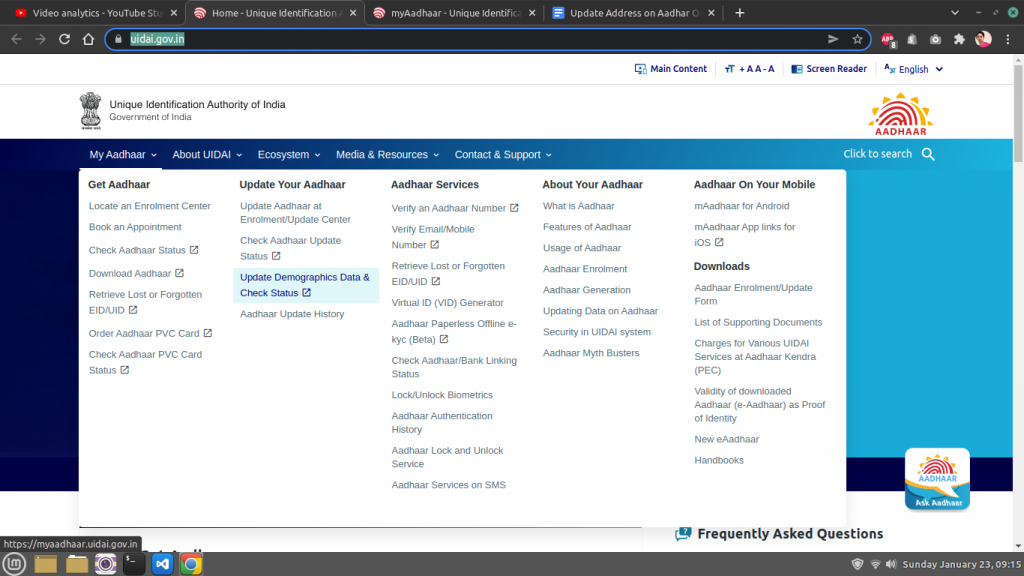This image depicts the official web page of the Unique Identification Authority of India (UIDAI), under the Government of India. The web page has a predominantly white background, with a blue gradient window located in the center. The gradient transitions from dark blue on the left to light blue on the right.

Within the blue area lies a prominent white rectangular box, horizontally oriented and containing various navigational options. These options are organized into distinct sections: "Get Aadhaar," "Update Your Aadhaar," "Aadhaar Services," and "About Your Aadhaar," followed by "Aadhaar on Your Mobile." Each section offers specific services listed in light gray text beneath the headings. For instance, under "Get Aadhaar," there are options such as "Locate an Enrollment Center," "Book an Appointment," and "Check Aadhaar Status."

At the top right corner of the page is the Aadhaar emblem, resembling a sun with red, swirling rays in the center, accompanied by the word "Aadhaar" in bold red capital letters: "AADHAAR." The overall layout is clean, designed for easy navigation and accessibility of essential services related to Aadhaar.